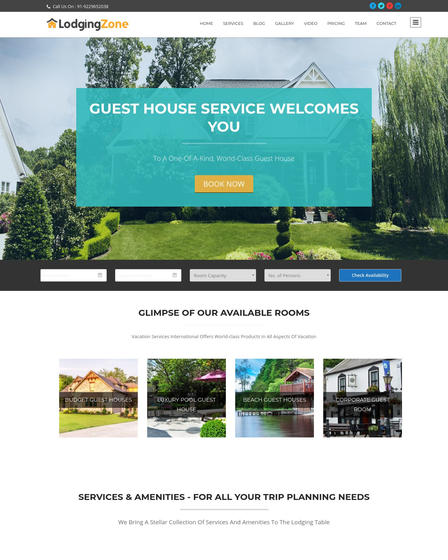The image showcases a web page belonging to a company named "Lodging Zone." The most prominent feature at the top of the page is a turquoise box with an inviting message: "Guest House Service welcomes you to a one-of-a-kind world-class guest house." Within this turquoise box, an orange "Book Now" button is visible, likely allowing users to initiate the booking process for various properties. 

Above this main section is a navigation bar offering links to sections such as Home, Services, Blog, Gallery, Video, Pricing, Team, and Contact, providing comprehensive access to the site's features.

Towards the bottom of the page, there are thumbnail images displaying different types of accommodations available. These include "Budget Guest Houses," "Luxury Pool Guest House," "Beach Guest House," and "Corporate Guest Room," each representing a diverse range of lodgings available for booking.

Overall, the web page appears to be a detailed and user-friendly platform for booking various types of guest houses curated by Lodging Zone.